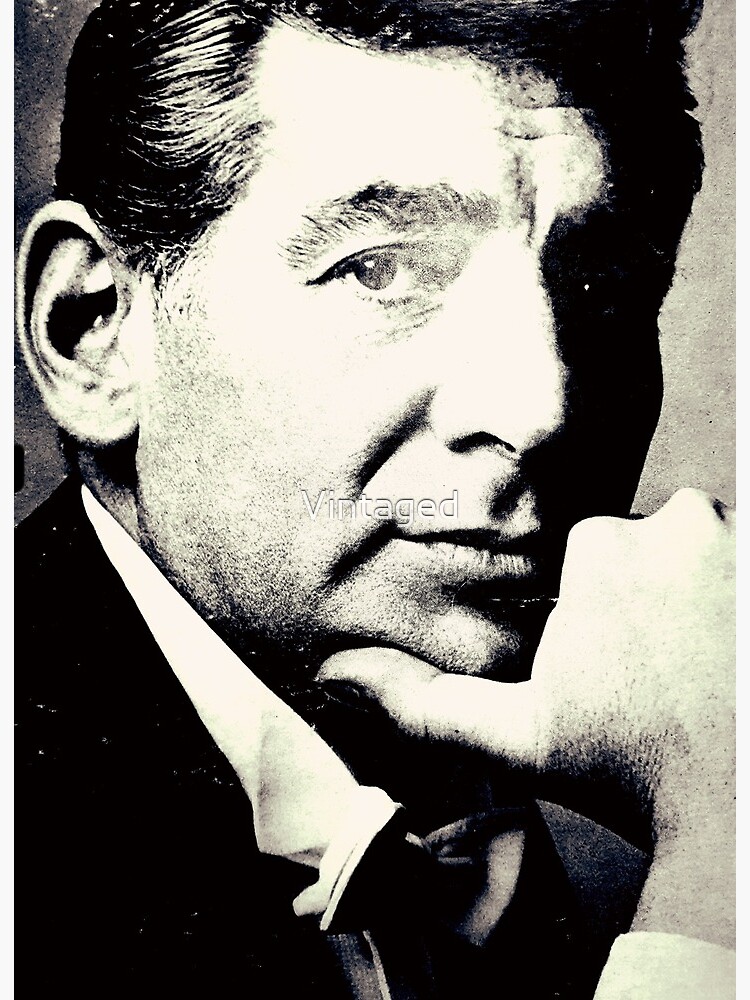This is a vintage professional black-and-white photograph of a man from the 1960s to 1980s, possibly a famous figure, perhaps even Jerry Lewis's sidekick. The image is a close-up, three-quarter profile portrait taken in a formal studio setting. The man has black hair and is wearing a suit with a white collar and a black bow tie. He is posing with his thumb under his chin and the rest of his hand covering part of his mouth, while looking straight at the camera with a slight smirk. Distortions and artifacts, such as flecks and abrasions, add a television fuzz-like effect to the photograph. His right eye appears slightly distorted, with areas of abrasion, and there is a shadow cast over his left eye, making it nearly black. Additionally, his eyebrows are bushy but also partially smudged, reminiscent of charcoal. The photograph features the word "vintage" in the middle, by his lips.